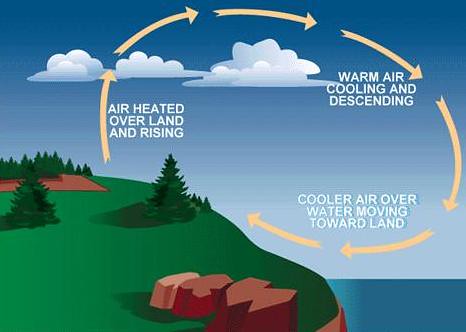This is a full-color, computer-generated diagram depicting the interaction between air, land, and water. The top portion of the image is dominated by a blue sky with three puffy white clouds. On the sky background, yellow arrows form a circular pattern, illustrating the flow of air. The arrows begin at a green grassy area on the left, rise up toward the right over the clouds, descend on the right side, and return leftward toward the land. The text, which is all in white uppercase letters, labels each segment of the air flow: "AIR HEATED OVER LAND AND RISING," "WARM AIR COOLING AND DESCENDING," and "COOLER AIR OVER WATER MOVING TOWARD LAND." 

At the bottom of the image, the green grassy area features a few pine trees and three rocks in the foreground. In the far distance of this grassy expanse, there is a brown dirt area with more trees visible. On the lower right-hand side, a blue rectangular section represents water. The diagram effectively illustrates the cycle of air movement and how breezes interact with land and water.